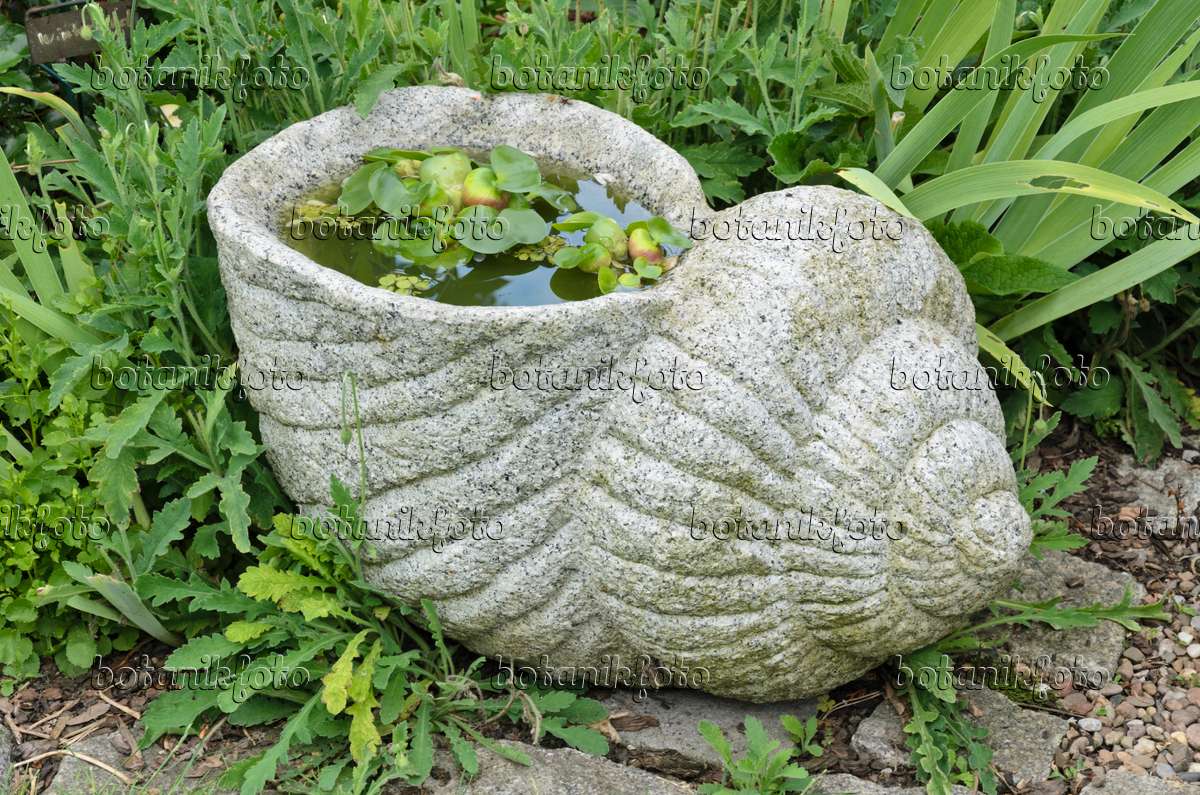This image is a detailed landscape-oriented color photograph capturing the serene scene of an outdoor garden. The central focus is on a unique bird feeder art piece designed to resemble a large concrete snail shell, which rests on its side with the tapered spiral pointing right. The shell is constructed from light gray concrete with speckles and recessed ridges mimicking the natural lines of a snail’s shell. The shell is open at the top and filled with murky dark green water.

Floating on the water's surface are several small aquatic plants and round-shaped fruits, which resemble small apples, suggesting the presence of nearby fruit trees. Surrounding the bird feeder, thick, leafy plants and green weeds fill the garden space, some with insect-eaten holes adding to the natural, untouched feel of the setting. Below the snail shell, the ground is adorned with a mix of small square dark gray paver rocks and diverse colored pea gravel, providing a stable base for the feeder. 

The overall scene is lush and full of life, with the natural imperfections such as weeds and insect-eaten foliage enhancing its authenticity. The photograph also contains a watermark reading "Botanic Photo," and is characterized by a style of photographic representationalism realism, meticulously detailing the textures and elements present in this charming garden vignette.